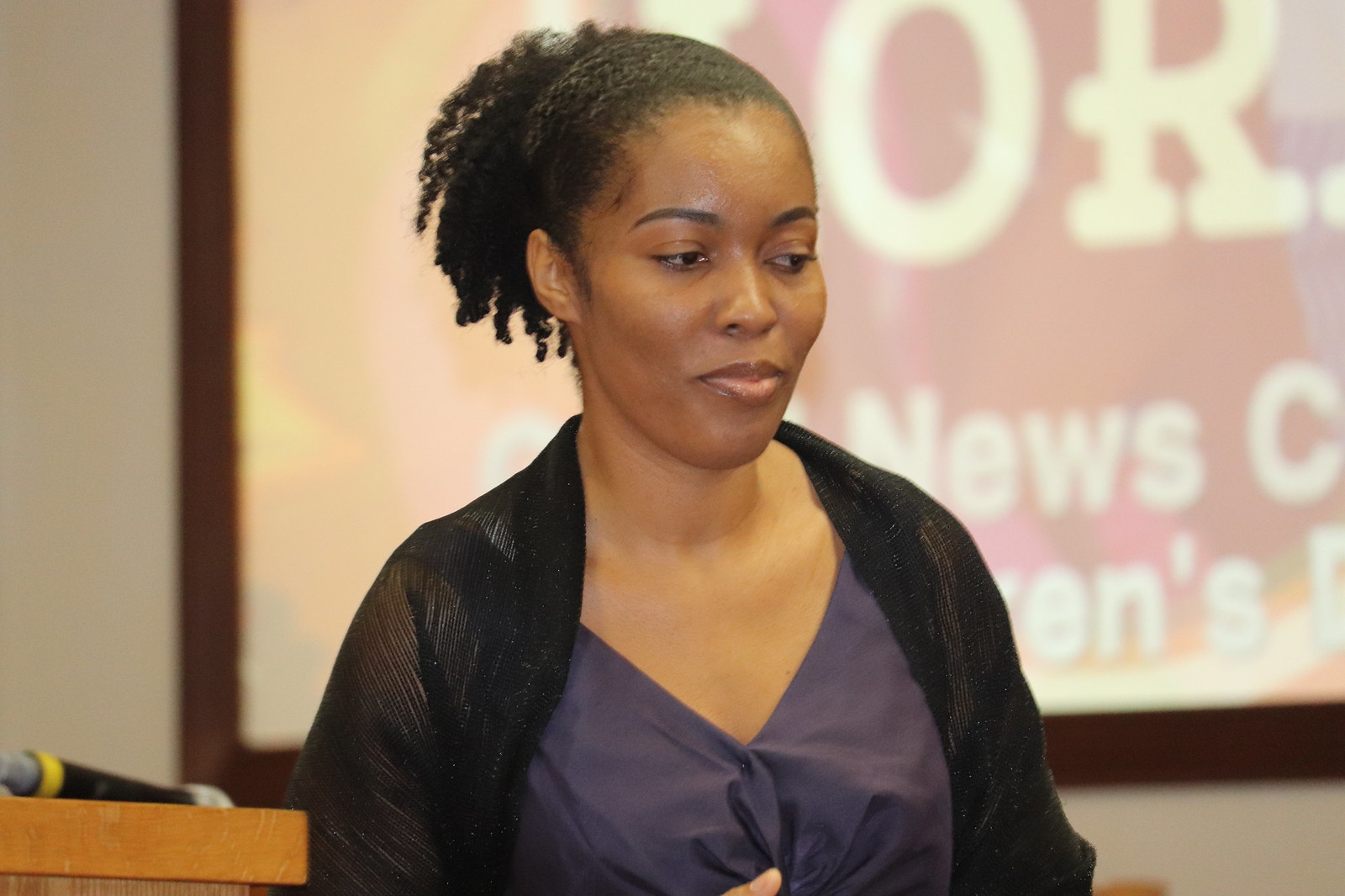The image features a young, attractive black woman seen from the mid-waist up in a medium close-up shot. She wears a purple dress paired with a sheer black cardigan. Her curly black hair is styled in a high ponytail. The woman appears contemplative, looking slightly downward, possibly at someone or something out of frame. To her right, but on the left side of the image, there's an unused microphone sitting on a light brown podium. Behind her, a projection screen displays a blurred slide with fragments of text that possibly include the words "News Center," and a partial phrase that might be related to children's content. The screen’s first visible word appears to start with "north," though only the letters O and R are clearly discernible. The background wall is a bit blurry but is discernibly white.